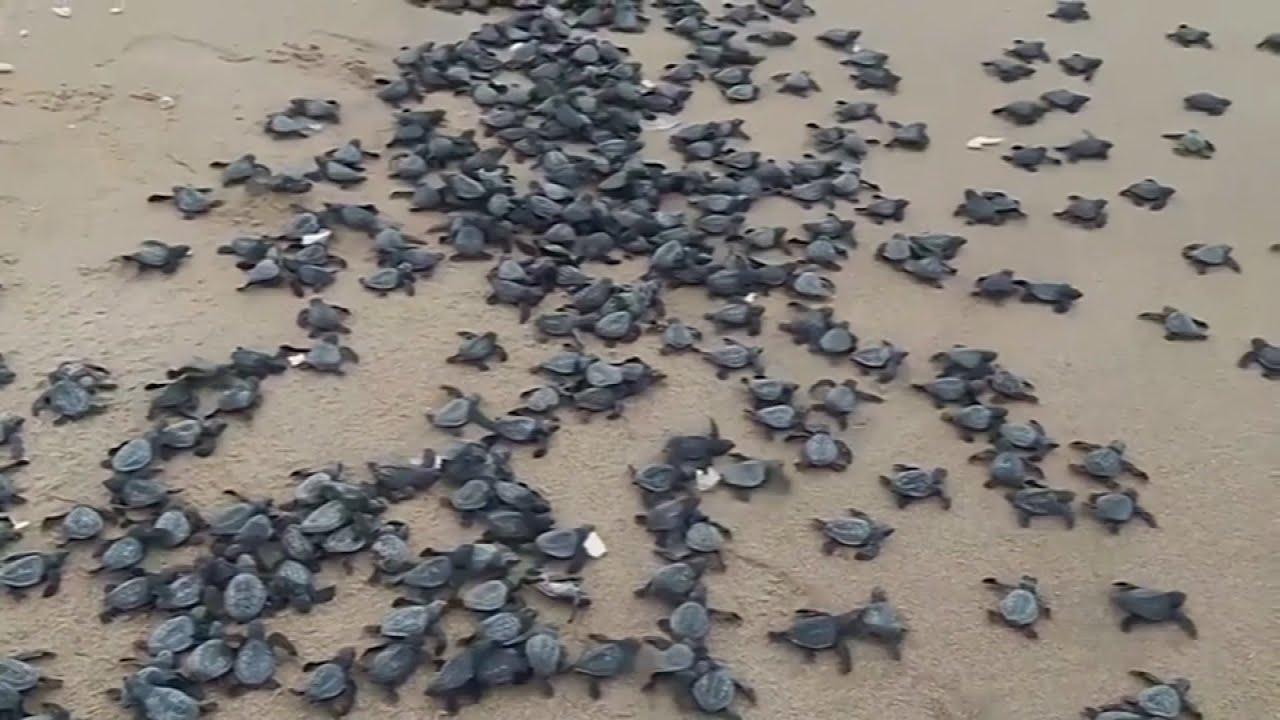This close-up, outdoor photograph captures an overcast beach scene, likely during the morning or evening, with wet, dark sand as the ground. The full-color, horizontally rectangular image shows dozens, possibly hundreds, of dark green to grayish sea turtle hatchlings, fresh from their eggs. The baby turtles are scattered across the beach, predominantly moving in a unified direction towards the upper right of the frame, likely heading to the ocean, which is not visible. Some of the turtles are climbing on top of each other, creating dense clusters, especially towards the upper part of the image, where it appears chaotic and tightly packed. Tiny footprints mark their paths in the sand, which is dotted with a few white shells. The photograph has a natural, unposed quality, suggesting it may have been taken by a professional photographer capturing this remarkable moment in nature.